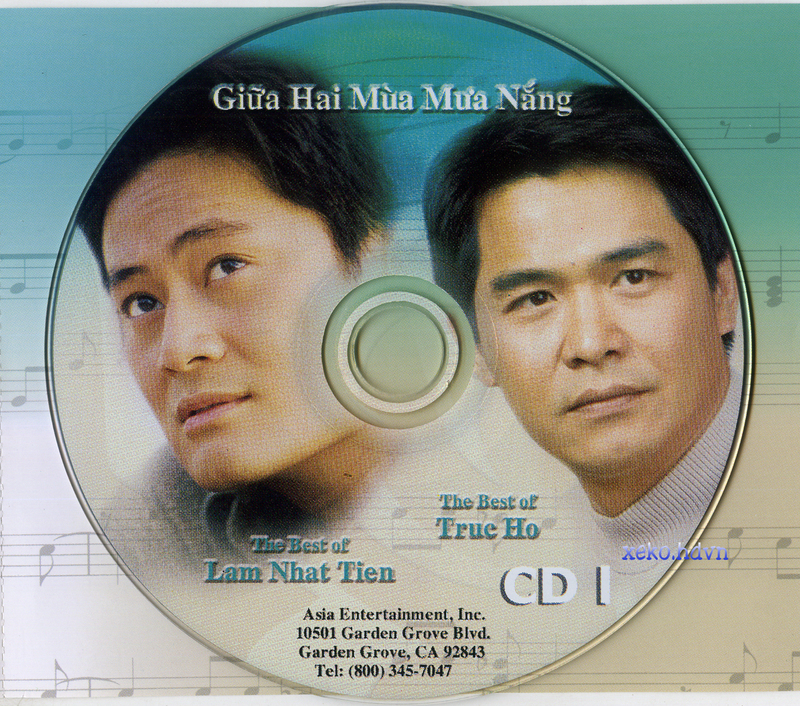This photograph depicts a CD with the label and text primarily in a foreign language, likely an Asian one. The backdrop of the image features a gradient that flows from blue at the top to brown and pink hues at the bottom, adorned with music bars and presumably music notes. The central focus is on the CD itself, which displays the faces of two men of Asian descent, both with dark hair and dark eyes, gazing off to the side. The CD features the text "The Best of Lam Na Tien" below one man's face and "The Best of Tru Ho" below the other. The CD is labeled "CD 1" and includes additional information: "Asia Entertainment Inc., 10501 Garden Grove Boulevard, Garden Grove, California, 92843, telephone 800-345-1047." There also appears to be a mention of a website, "exeko.htvn," suggesting this is part of a media promotion package.